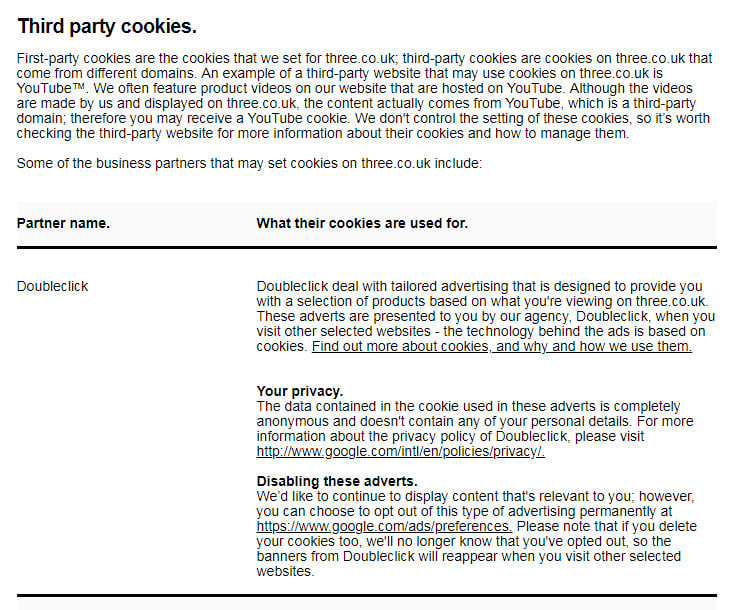This image depicts a comprehensive information page about third-party cookies on 3.co.uk. The layout is clear and organized, providing users with detailed explanations in plain, informative language. 

At the top of the page, a bold, straightforward title introduces the topic of third-party cookies. Beneath this, smaller text explains the distinction between first-party and third-party cookies: 

"First-party cookies are set by 3.co.uk, whereas third-party cookies originate from different domains. For instance, YouTube, a third-party website, may use cookies on 3.co.uk. We frequently feature product videos hosted on YouTube. Although these videos are created by us and displayed on 3.co.uk, they are technically from YouTube, a third-party domain. Consequently, you may receive a YouTube cookie. We don't control the settings of these cookies. For more information on third-party cookies and how to manage them, please check the third-party website."

Below this explanatory section, with a subtle gray background, the page outlines some business partners that may set cookies on 3.co.uk. There is a bold vertical line separating the partner's name on the left from the purpose of the cookies on the right. For example, under the heading “DoubleClick,” it states:

"DoubleClick cookies are used for table advertising, aiming to offer you product selections based on your activity on 3.co.uk. These adverts are presented by our agency and may appear on other selected websites. The technology behind these ads and their cookies enhances your browsing experience. Find out more about cookies, why and how we use them."

Further down, sections titled "Your Privacy" and "Disabling These Adverts" provide additional explanations on user privacy and options for managing ad preferences.

A horizontal black line runs from left to right at the bottom of the page, offering a clean separation from the other segments, ensuring a neat and professional presentation.